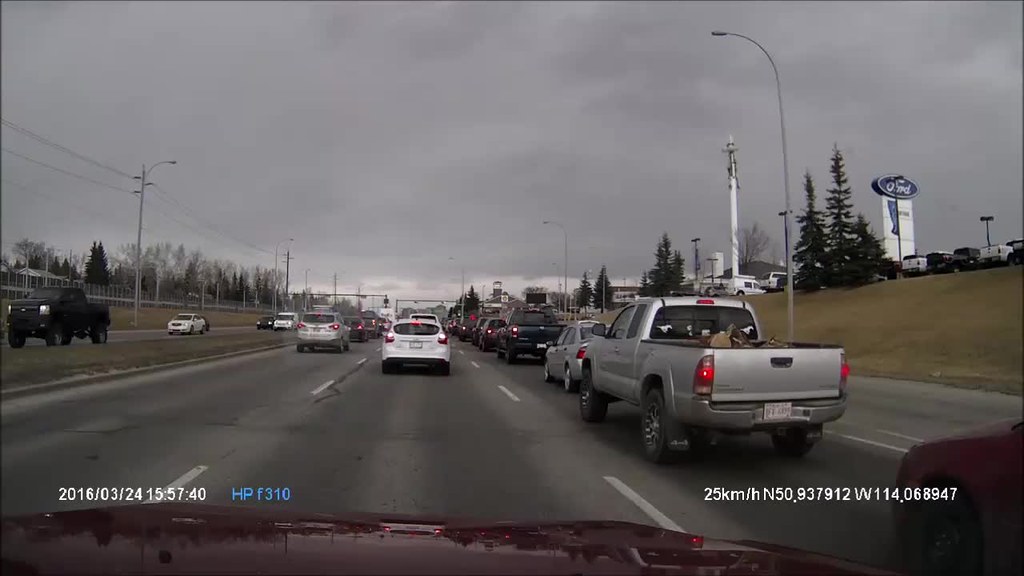A photo captures a bustling three-lane highway on a cloudy late afternoon or early evening, hinting at imminent rain. Traffic flows steadily in both directions, with vehicles moving swiftly, avoiding any congestion. Prominently, a silver truck hauling an unspecified load is noticeable, along with a white sedan in the middle lane and a silver SUV. Heading in the opposite direction, a black truck and several sedans trail slightly behind. The highway is flanked by trees on both sides, adding a natural contrast to the urban setting. Along the right side of the image, a car dealership, identified by vehicles neatly lined up, becomes visible. A blue and white Ford logo stands out, indicating the dealership's brand. The image suggests a chilly day with a slight chance of sleet.